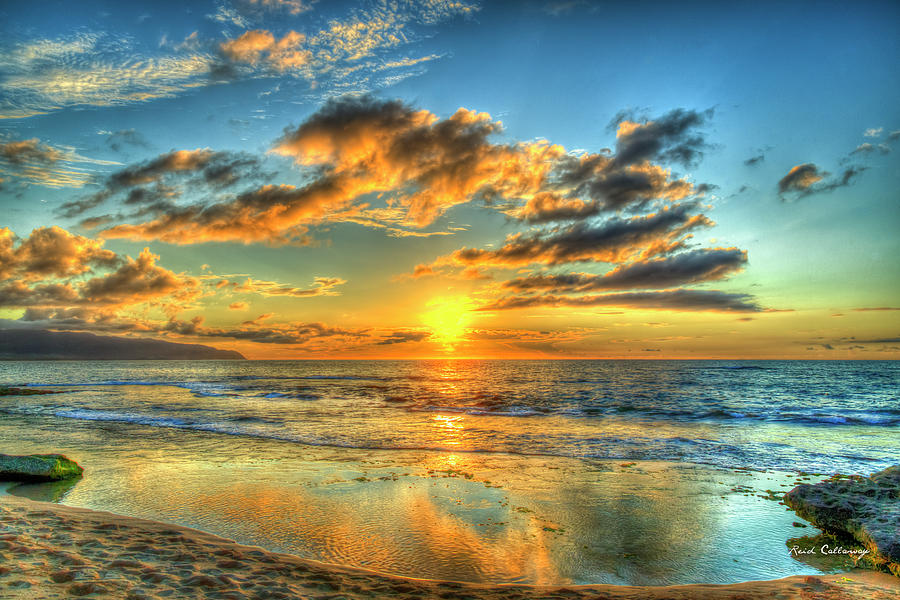This stunning high-definition photograph captures a tranquil ocean sunset at the beach. The scene is vibrant, with the sun just above the horizon, casting a rich, golden glow across the sky and the water. Wispy clouds are tinted in shades of gold, orange, and umber, with some areas appearing gray due to the shadows. The sky is a deep blue, gradually transitioning to golden hues as it meets the shimmering water below. Rolling waves gently reach the shore, with the sandy beach visible in the lower left-hand corner, gradually narrowing to the right and appearing darkened and shadowy. The sun’s golden reflections dance upon the surface of the ocean, adding to the serene atmosphere. In the lower right corner of the photo, the watermark “Reid Calloway” is delicately inscribed in fine, cursive white text. This exceptionally detailed image exudes a peaceful, relaxing ambiance, capturing the timeless beauty of a beach sunset.